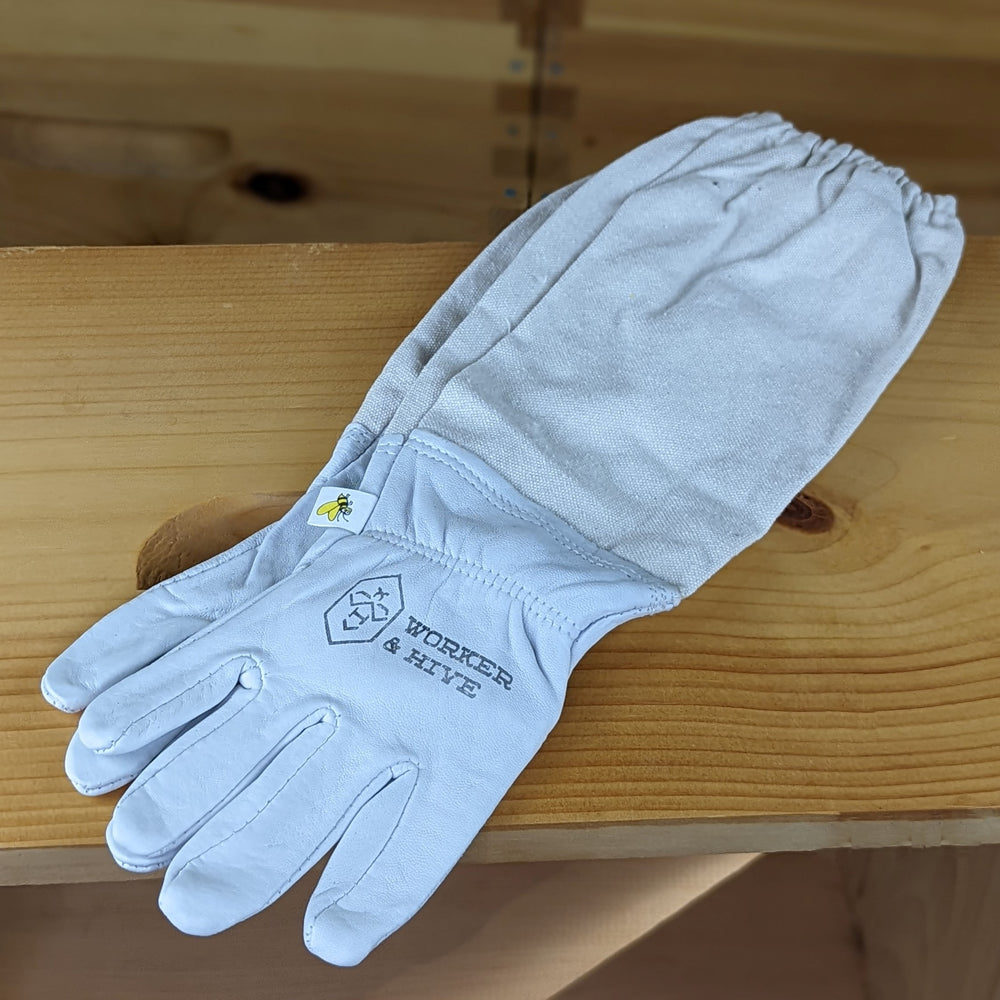The image captures a vertical photograph of a pair of beekeeping gloves, displayed on a natural-colored wooden plank, possibly a walnut 2x10 or 2x12 board. The gloves, which are overlapping one another, are made from a leathery material in a light blue-gray hue. They are characterized by their long sleeves extending up to the elbows and feature elastic cuffs for a secure fit around the arms. Each glove is marked with a hexagon-shaped logo that reads "WORKER & HIVE" in all capital letters, accompanied by a small white tag on the left side of the top glove. This tag includes a picture of a yellow and black bee, adding a touch of authenticity to their beekeeping purpose. The photograph as a whole shows the simplicity and utilitarian design of these essential protective gloves against a wooden background that complements their practical elegance.